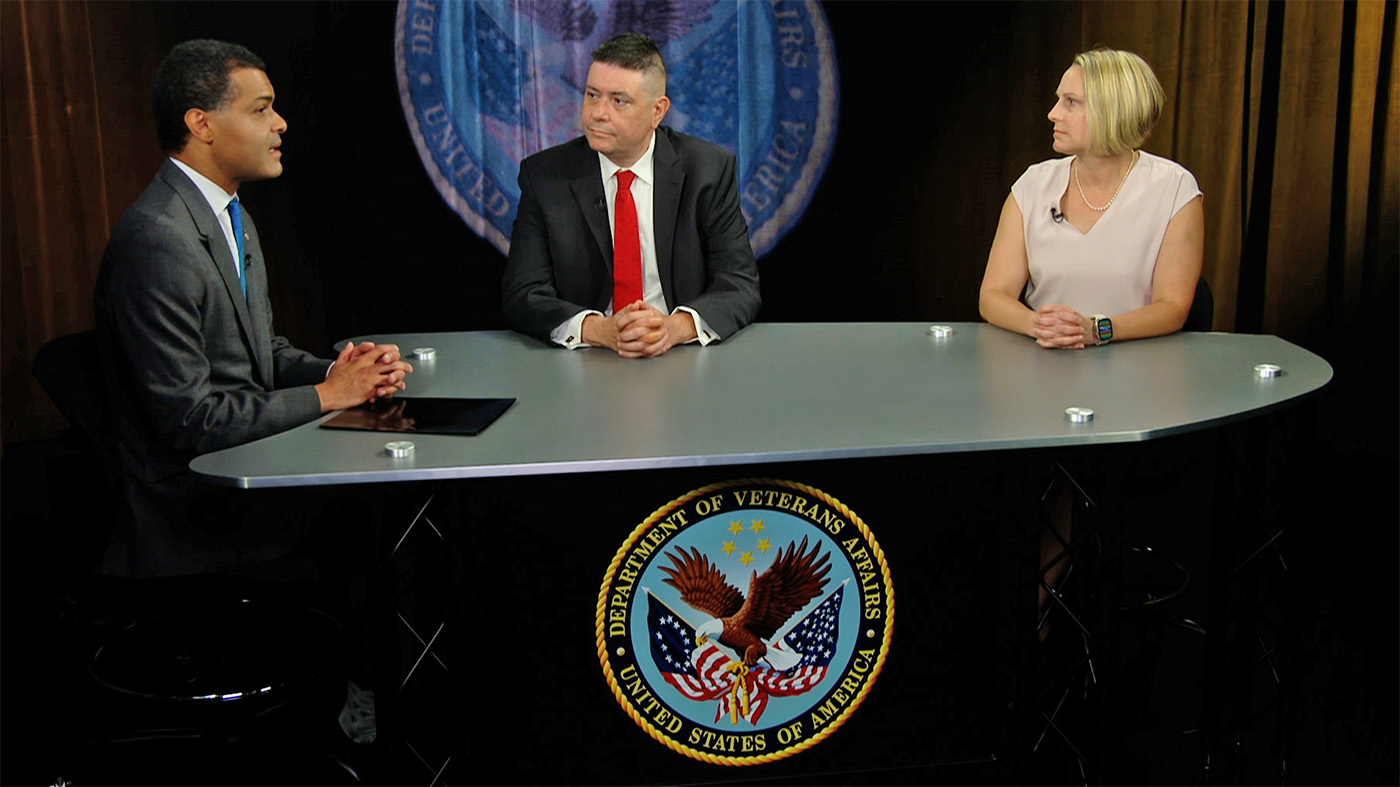The image depicts an intense moment between three individuals engaged in a political debate, with a clear focus on the Department of Veterans Affairs. The setting features a sleek, gray desk adorned with a plaque that reads "Department of Veterans Affairs, United States of America," framed by a prominent American Eagle gripping two American flags. 

Seated at the table are three people dressed in professional attire: a dark-skinned African American man with black hair on the left, a dark-haired Caucasian man in the middle, and a blonde Caucasian woman on the right. The woman wears a pearl necklace and a casual blouse, and it is noteworthy that she is blind. Both men sport suits and ties. Their fingers are interlocked and resting on the table, exuding a sense of seriousness. 

Everyone is sitting upright, and the white male and the female are attentively looking towards the African American man, who appears to be speaking. The atmosphere is formal, underscored by the United States insignia on the wall behind them, further emphasizing the gravity of their discussion.